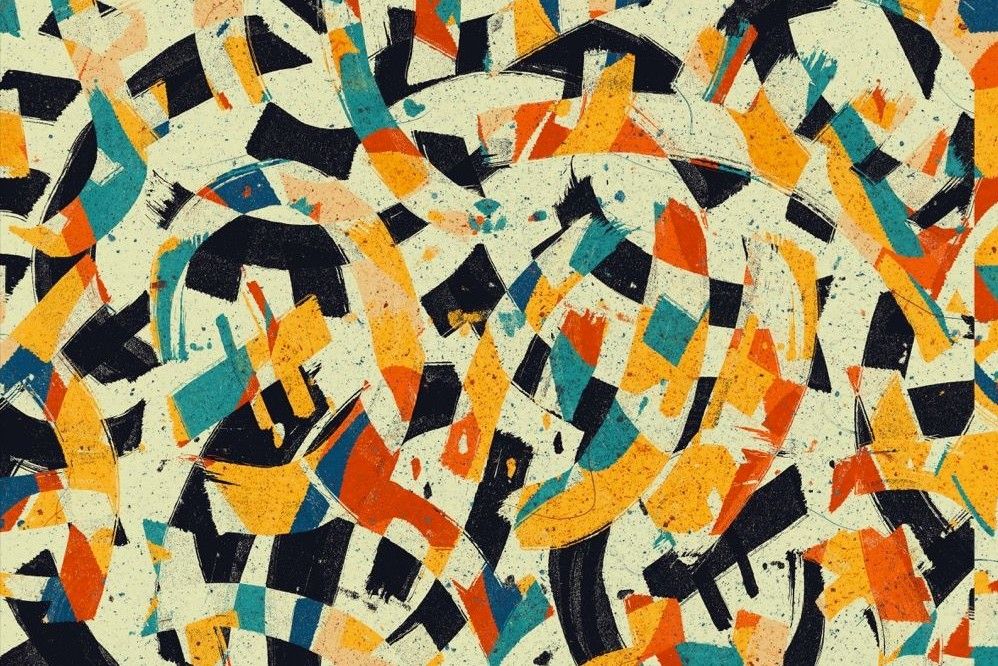The image is an abstract painting featuring a vibrant, chaotic array of shapes and colors. Predominantly, it showcases a repeating pattern of squares, rectangles, and triangles in hues of yellow, green, black, red, blue, and orange. The artwork also includes paint strokes and splotches of various colors set against an off-white background, adding an additional layer of texture and depth. The composition incorporates both solid blocks of color—like blue and black squares—and more fluid, curved lines, creating a balance of blocky and curvy elements. Despite its apparent lack of uniformity, the painting is visually cohesive, displaying a unique checkerboard-like quality interspersed with dynamic, abstract forms.